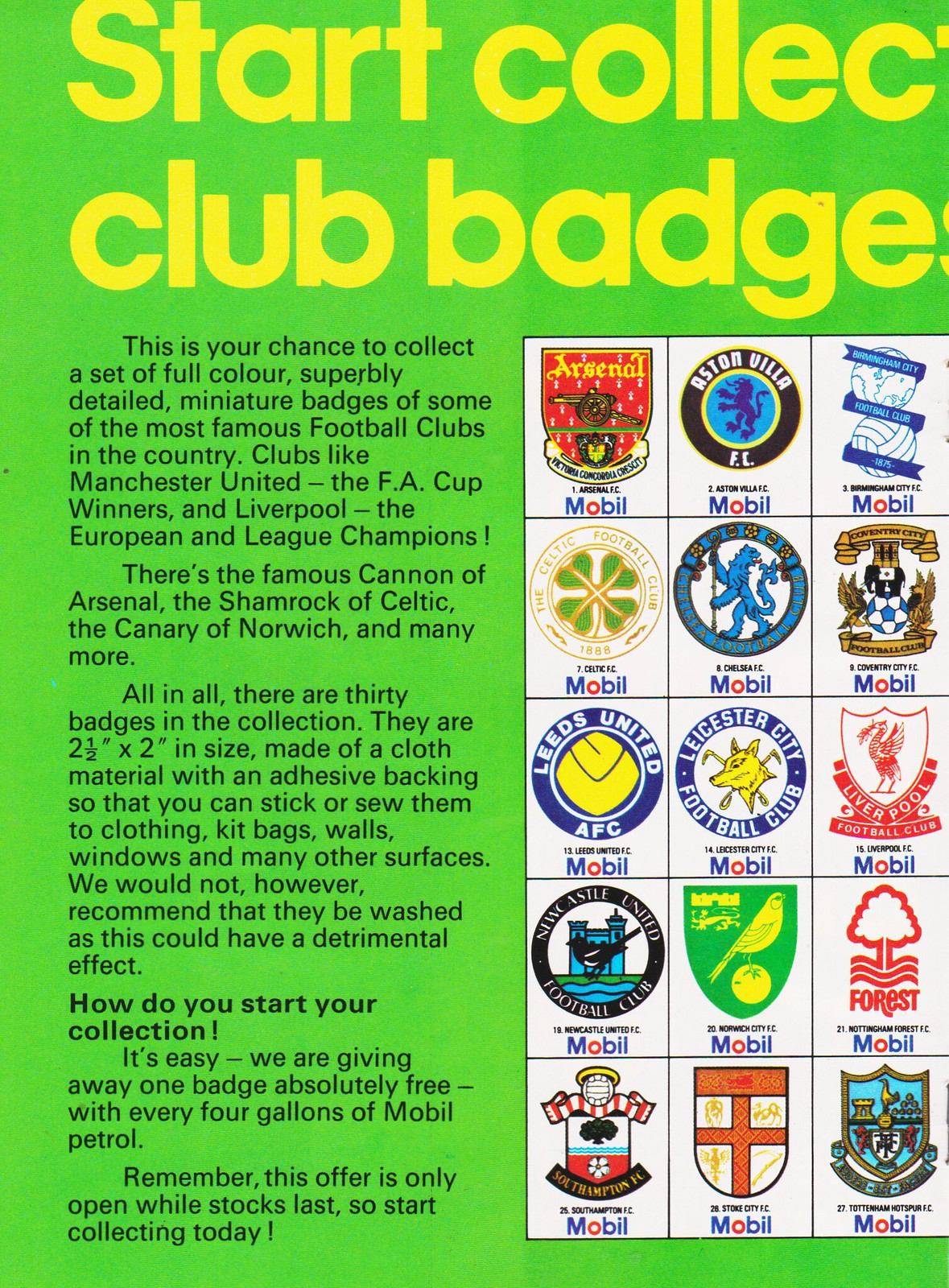This vibrant neon green poster invites enthusiasts to "Start Collecting Club Badges" with bold, yellow lettering at the top. Displayed in white, there are 15 detailed images of miniature badges on the right side, representing some of the most famous football clubs in the country, such as Manchester United (FA Cup winners) and Liverpool (European and league champions). The collection boasts 30 badges in total, showcasing iconic symbols, including the Canon of Arsenal, the Shamrock of Celtic, and the Canary of Norwich. Each badge is two and a half by two inches in size, made from cloth material with an adhesive backing allowing them to be easily stuck or sewn onto various surfaces like clothing, kit bags, walls, and windows. However, it is advised not to wash them as this may cause damage. Text on the left part of the poster explains how you can kickstart your collection: earn a free badge with every four gallons of Mobile petrol. Note, this offer is limited while stocks last, so start collecting today!